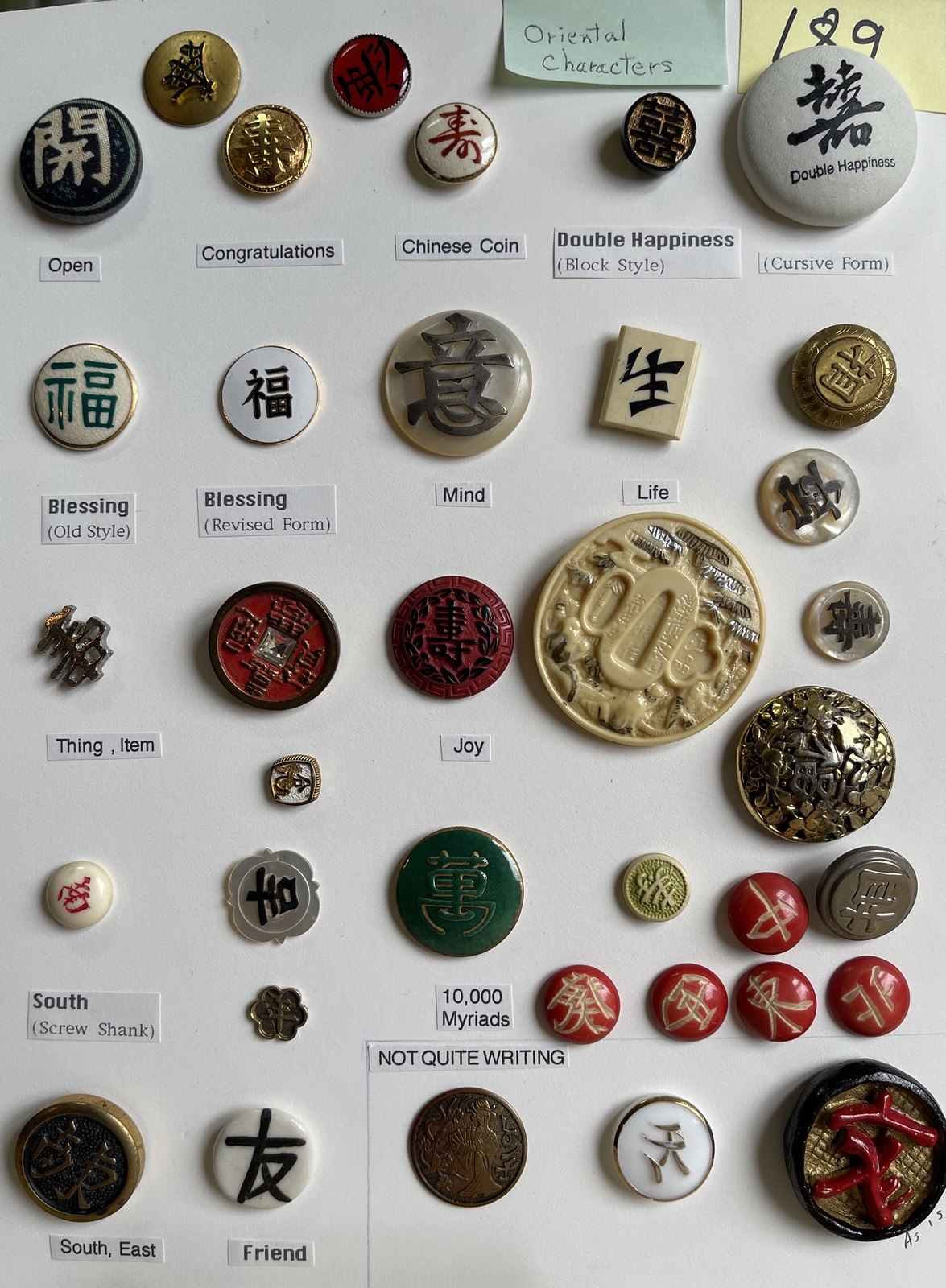The image displays a white poster board adorned with various oriental buttons and stones of differing colors, sizes, and styles. At the top right corner, a green sticky note with handwritten text reads "Oriental Characters." The buttons and stones, primarily in black, red, white, green, and gold, are carefully arranged across the board. Each button or stone is accompanied by small white labels with black lettering that explain their meanings. Some of the inscriptions include: "open," "congratulations," "Chinese coin," "double happiness," "blessing," "mind," "life," "thing/item," "joy," "south," "ten thousand myriads," "southeast," and "friend." The detailed arrangement and accompanying labels suggest a thoughtful presentation of various Chinese characters, their interpretations, and their artistic styles.